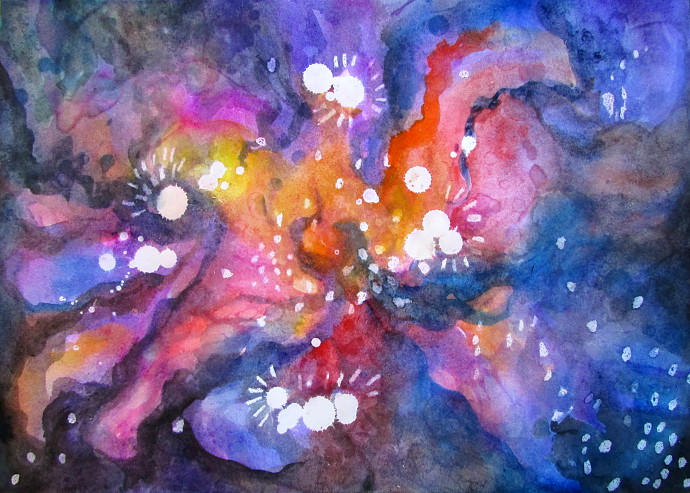This image showcases an abstract watercolor painting with a distinctly 90s aesthetic. The composition is a swirling medley of colors including vibrant pinks, purples, blues, whites, browns, oranges, and reds. The left side of the painting is dominated by various shades of blue, from light to dark, while the right side features more black and grayish tones. Scattered throughout the entire canvas are tiny white circles, totaling around 50, with about 10 to 15 medium-sized ones concentrated in the center. The central area is also infused with warm hues of orange, pink, and yellow. The overall effect is reminiscent of tie-dye patterns or the swirling colors of the northern lights, though it remains devoid of any concrete shapes, evoking more of a fluid, almost aqueous ambiance.